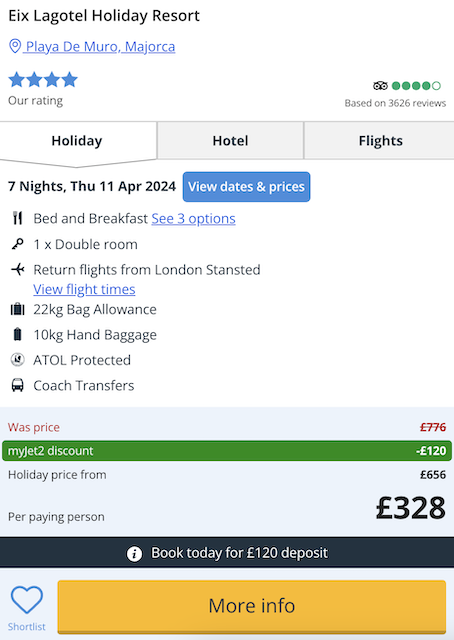The image is a vertical screenshot of a holiday resort booking page, formatted for mobile but slightly wider, likely tailored for an iPad display, characterized by a predominantly white background. 

In the top left-hand corner, the resort is identified as "EIX Lag Hotel Holiday Resort," located in Playa de Muro, Mallorca, and rated with four blue stars. The page features an R-rating and three main tabs underneath labeled "Holiday," "Hotel," and "Flights," with "Holiday" currently highlighted in white while the other tabs are in gray. 

Detailed information about the hotel package is visible below the tabs. The offer includes a stay of seven nights starting Thursday, 11th April 2024. A prominent blue button is labeled "View dates and prices." The package includes bed and breakfast with three available options, featuring one double room, return flights from London Stansted, specified flight times, a 22-kilogram checked baggage allowance, a 10-kilogram hand baggage allowance, ATOL protection, and coach transfers.

The page also highlights a discount: the original price of £776 has been reduced by £120 thanks to a MyJet 2 discount, bringing the total to £656. This reduction translates to a price of £328 per paying person. Additionally, there is an option to secure the booking with a deposit of £120. At the bottom, a yellow button labeled "More Info" is available for additional details.